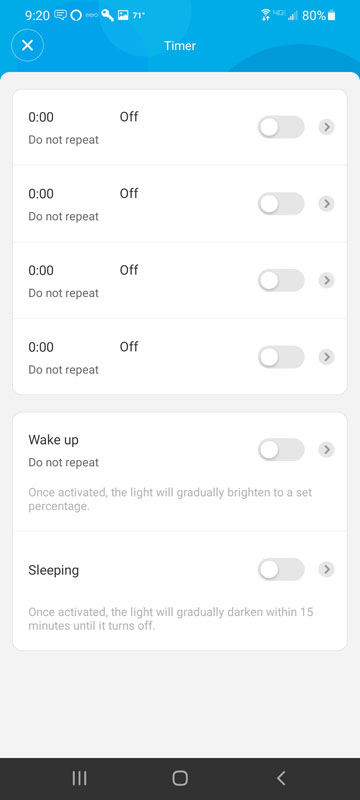The image depicts a timer application displayed on a smartphone. The interface features a prominent blue header adorned with light, curvy, and darker graphic elements in varying shades of blue. The clock shows "9:20." Icons for a speech bubble, key, photo, Wi-Fi, and a signal indicator with two bars, along with an 80% battery icon, are present at the top.

On the left side of the header, there is an 'X' inside a circle. Adjacent to the timer display, labeled "Timer," is a white overlay with a subtle drop shadow, housing four identical settings sections. Each section includes:
- 0.0
- 0 minutes, 0 seconds
- An "off" slider switch with "Do not repeat" indicated.

These sections are repeated four times. Below these, options labeled "Wake Up" and "Do not repeat" are also switched off. A description under "Wake Up" notes that once activated, the light will gradually brighten to a specified percentage.

Further down, the "Sleeping" option, also set to off, states that once activated, the light will gradually darken over 15 minutes until it turns off. The black navigation bar at the bottom displays three buttons.

The overall impression from the image is that the timer app is inactive, with all functionality turned off and no custom settings applied. The most noteworthy visual element is the blue header with its assortment of circular graphics, albeit unremarkable in design.